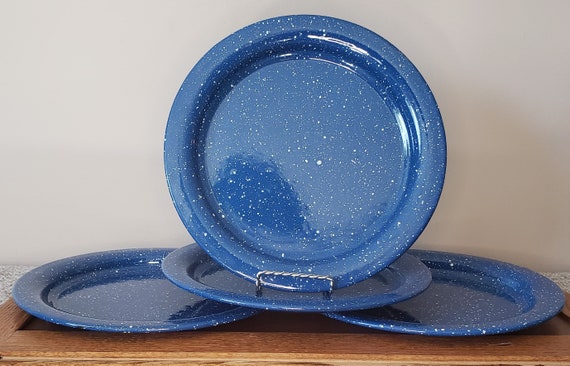This indoor photograph captures a rectangular image, approximately four inches wide by three inches high, showcasing a serene, minimalistic setting. A light gray painted wall serves as a backdrop, extending down to about three-fourths of the photo where it meets a white stone countertop speckled with gray. Resting on the countertop is a brown wooden surface. 

Centered on this wooden surface are four blue enamel plates adorned with subtle white specks resembling delicate paint splatters. Arranged thoughtfully, two plates lie flat side by side, while a third plate rests atop them, featuring a raised silver handle, suggesting it doubles as a platter. The fourth plate is positioned upright, supported by a metallic holder, which nestles it gracefully against the wall. This standing plate mirrors the color and delicate speckled pattern of its companions, completing the harmonious composition.